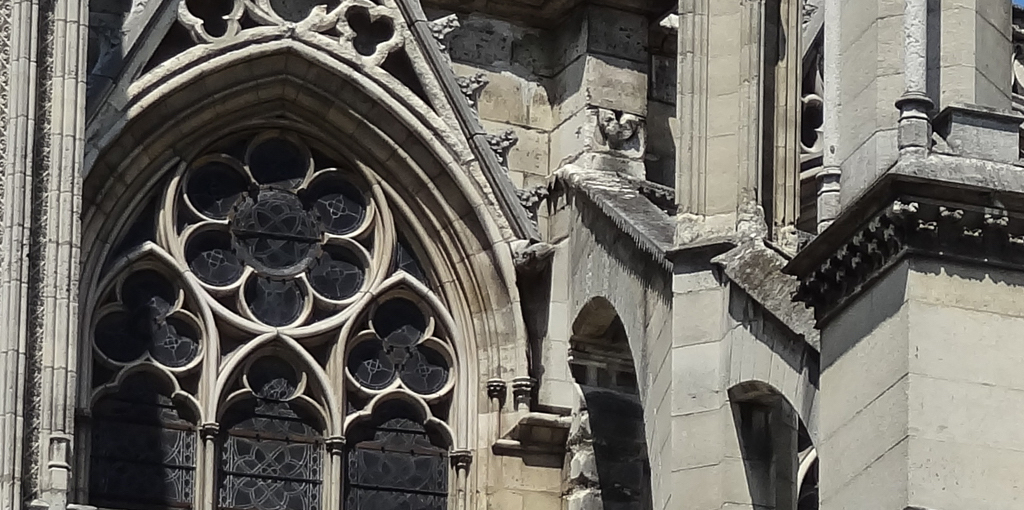The image captures a detailed close-up of the exterior of what appears to be a historic church or cathedral, characterized by its light gray stone architecture. Central to the photograph is an intricately designed arched window, featuring three smaller arches within it and a circular stone pattern resembling a flower burst in the center. The window glass appears opaque, possibly due to the way the photo is taken. Surrounding the window, there are additional architectural features including archways sloping towards the camera and at least two pillars, one on the far left and another on the right, contributing to the structure's support. The overall scene, with its combination of dark and light contrasts, suggests the grand, yet somber, ambiance typical of such monumental buildings found in bustling city centers.